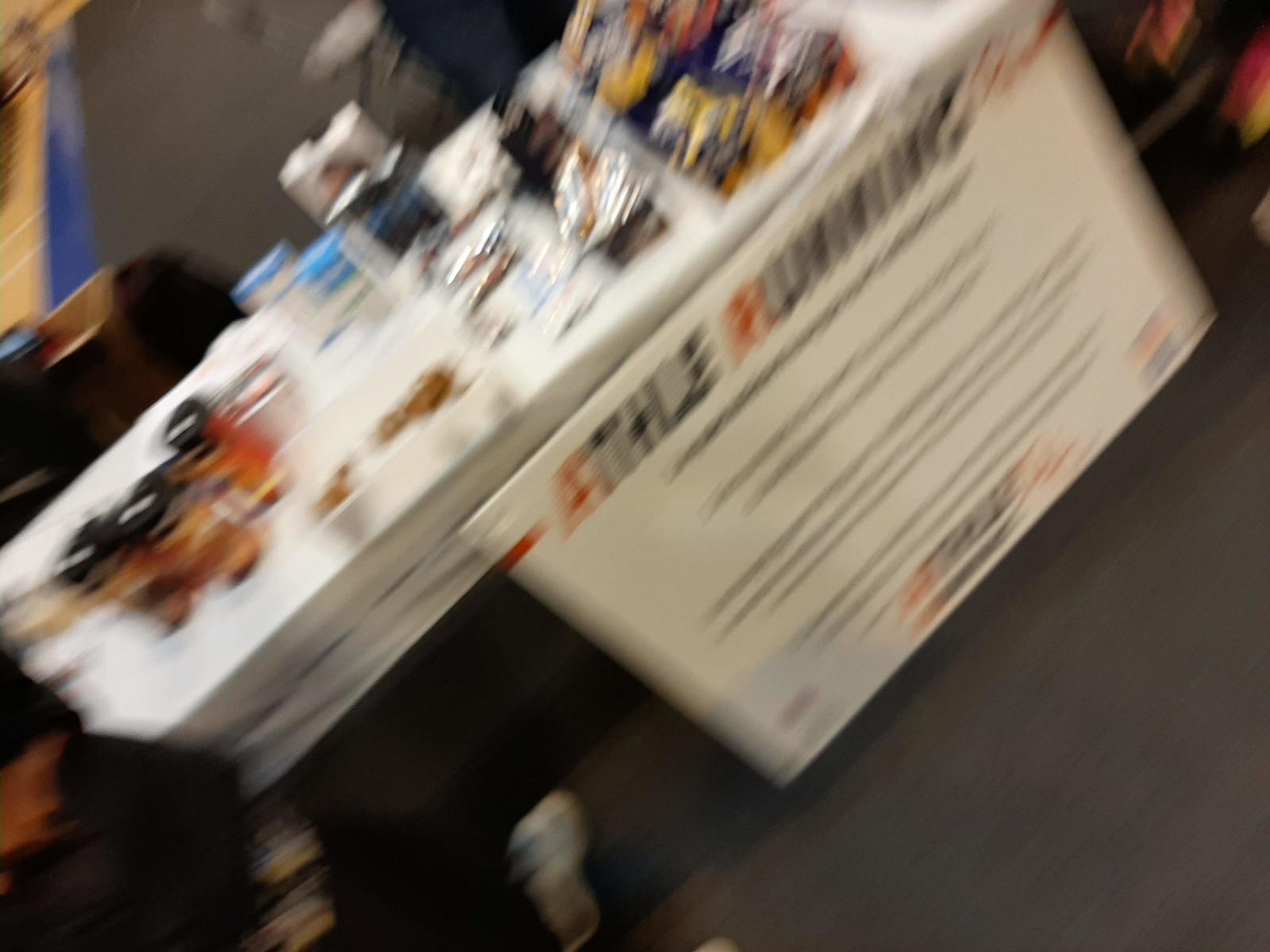This photograph, though blurry, offers a glimpse into a bustling scene. Central to the composition is a white sign adorned with black and red lettering, prominently featuring the word "running". The sign is affixed to the edge of a table draped in a crisp white tablecloth. Despite the lack of focus, the table appears to be laden with various products, including what seems to be canisters and energy bars, likely catering to an event or store display related to running. The overall impression is that the image may have been taken unintentionally, perhaps in haste or by an accidental press of a camera button, capturing an unplanned, candid moment.